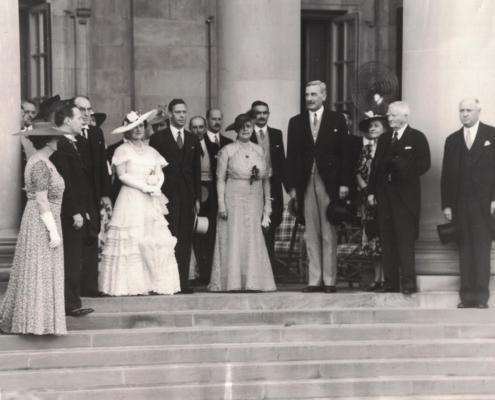This black and white photograph, likely from an earlier era, depicts a group of about 20 individuals standing on the wide stone steps of a grand, government-like building characterized by its white stone columns and embellished architecture. The men and women, dressed in formal and elegant attire, are arrayed at various levels on the staircase. The women don long, fancy dresses with matching hats and gloves, while the men wear formal black suits and top hats, which they hold by their sides. One man deviates slightly with cream-colored pants. Notably, a tall man in a suit stands next to a shorter woman with a flower adorning her chest, both suggested to be central figures, possibly indicating a special occasion such as a wedding. Another couple nearby includes a woman in a frilly white dress holding a flower and a man in a suit. Behind the group, wicker chairs with plaid-patterned cushions provide a glimpse into the decor of the era. The meticulous detailing of attire and the grandiose setting of the building suggest an event of significance captured in this timeless photograph.